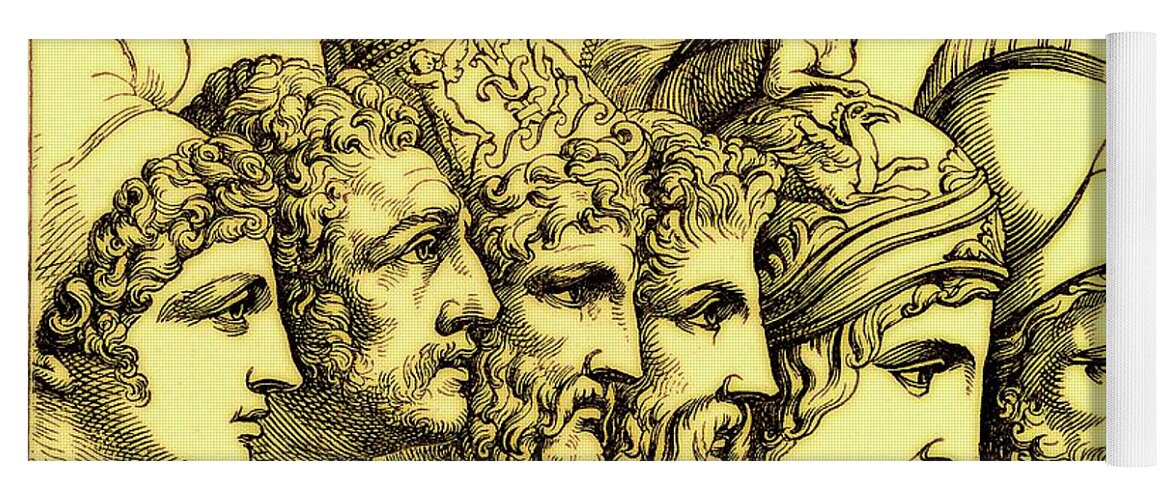This detailed black and yellow horizontal illustration, reminiscent of ancient Greek art, depicts side profiles of six figures believed to be prominent men from the Trojan War, such as Odysseus, Agamemnon, and Hector. The artwork, resembling pencil or ink drawings akin to the elaborate style of historical figures on currency, has a predominantly light green or yellow tone with white accents. From left to right, the first man is clean-shaven with short, curly hair and wears a small white hat. The second figure, with a weathered face, sports a thin mustache and beard. The third man, with his head slightly tilted forward, features short, curly hair and an ornate helm decorated with a cherub and a sword, showcasing a detailed beard and mustache. The fourth profile shows a man with a long, thin nose, a thick mustache, and wavy hair. The fifth head is partially obscured, revealing only hair beneath a helmet adorned with a dragon-bird motif. The sixth partial figure displays hair flowing from a helmet with a noticeable crack on top. Each figure’s intricate curly hair and facial details contribute to the richly textured, historically evocative scene on what appears to be a yoga mat.